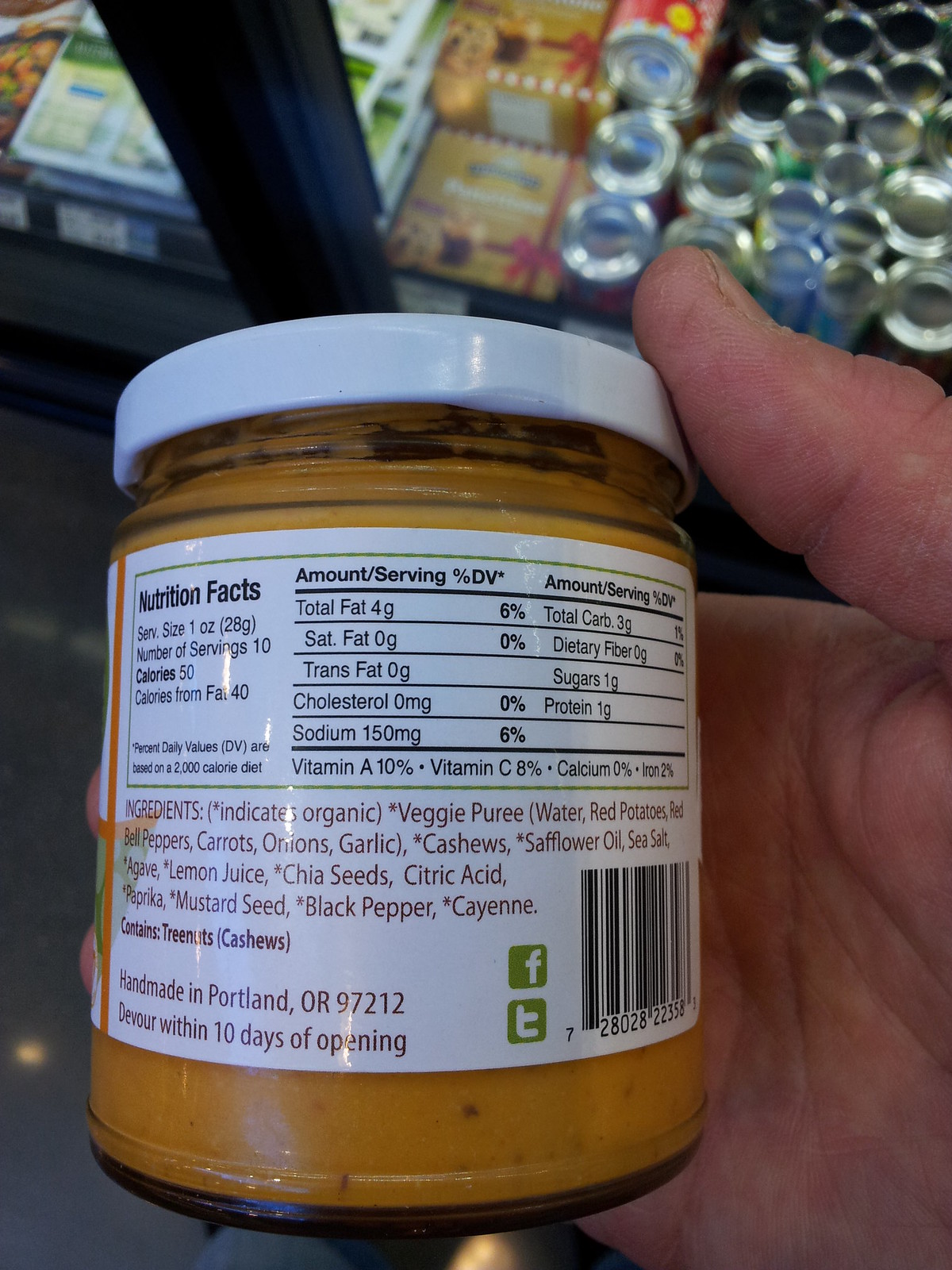A small glass jar with a white cap, containing a handmade food product, possibly a veggie puree. The label lists the ingredients as: veggie puree, water, red potatoes, red bell peppers, carrots, onions, garlic, cashews*, sunflower oil*, sea salt, agave, lemon juice, chia seeds*, citric acid, paprika, mustard seed*, black pepper*, and cayenne. The product contains tree nuts, specifically cashews, and is handmade in Portland, Oregon. The jar must be consumed within 10 days of opening. 

On the label, there are symbols including a barcode, a green Facebook logo, and Twitter's old logo represented as a lowercase 't' within a green-bordered box. Though the initial impression might suggest it could be baby food, the consumption recommendation suggests otherwise.